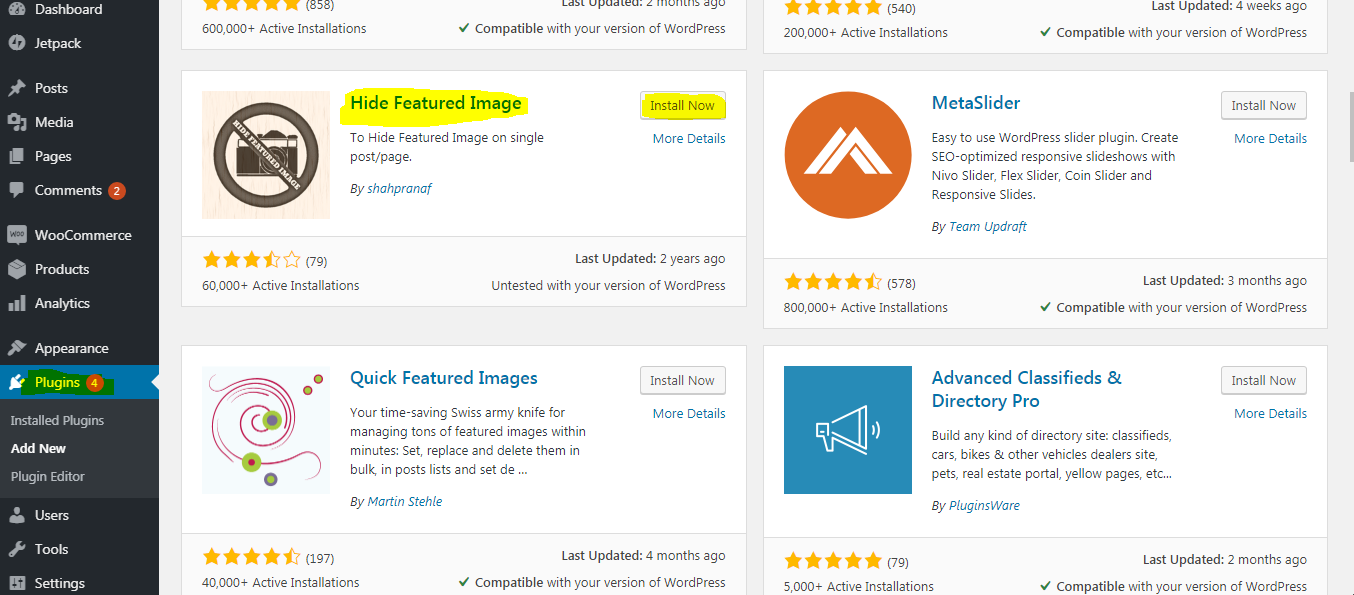This screenshot depicts a section of a website's admin page, specifically focused on available add-ons. On the left side of the image, there is a vertical, black-colored navigation panel listing various categories, including Dashboard, Jetpack, Posts, Media, Pages, Comments, Web Commerce, Podcasts, Analytics, Appearance, and Plugins. The Plugins category is both highlighted in green and currently selected, indicated by a blue highlight.

To the right of the navigation panel, there is a section displaying four available plugins. The first plugin, titled "Hide Featured Image," features a thumbnail image on its left, an "Install Now" button, a user rating positioned in the bottom left corner of the plugin description, and information on the last update in the bottom right corner. The second plugin, "Meta Slider," also includes a thumbnail to its left, alongside an "Install More Details" button on the right, a rating in the bottom left corner, and update information in the bottom right. Two additional plugins are listed below these, continuing the same layout format.